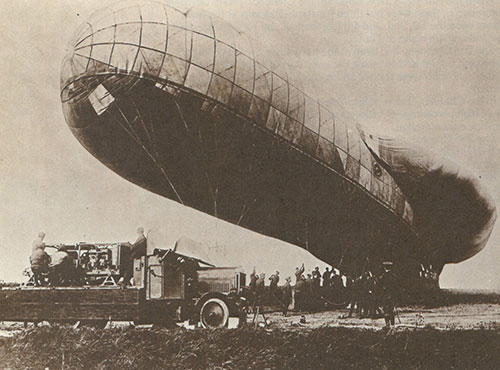In this vintage sepia-toned black and white photograph, we see an early depiction of a zeppelin, possibly the Hindenburg, either landing or preparing for launch. The zeppelin dominates the scene, with the nose slightly more elevated than the tail, indicating some slack in the anchoring ropes. A multitude of small, indistinct figures—men in old-timey attire with caps—are holding onto the numerous guy wires securing the zeppelin, making them look like they're pulling down a giant balloon. An old fire truck with distinctive white-rimmed tires stands in the foreground, its bed occupied by four men. The ground is a mix of grass and dirt, and there appears to be a raised platform or stage area beneath the zeppelin with large boxes, although their purpose is unclear. The blimp itself is smooth, with dark lines creating a rectangular grid pattern along its side, and its underside is cloaked in shadow. The sky forms the backdrop, enhancing the historical atmosphere of this early aviation endeavor.